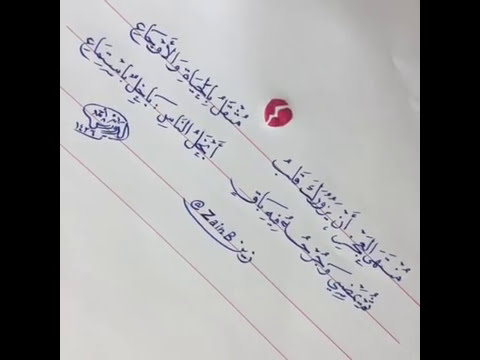The image is a close-up photograph of a white or off-white paper featuring blue Arabic script written on a series of lines, which are slanted from the top left to the bottom right, resembling the orientation of musical staff lines. Above the Arabic writing, there is a prominent red logo that resembles a broken heart with a jagged white lightning bolt or line dividing it in half. The Arabic script contains characters with numerous perpendicular lines and dots, with some letters extending below the ruled lines. At the very bottom of the script, the Roman alphabet is used to spell "Zain B," suggesting a social media handle or a name, presented as "Z-A-I-N B." The overall composition of the photograph has a tilted angle, giving the appearance that the entire content is slanting downward diagonally.